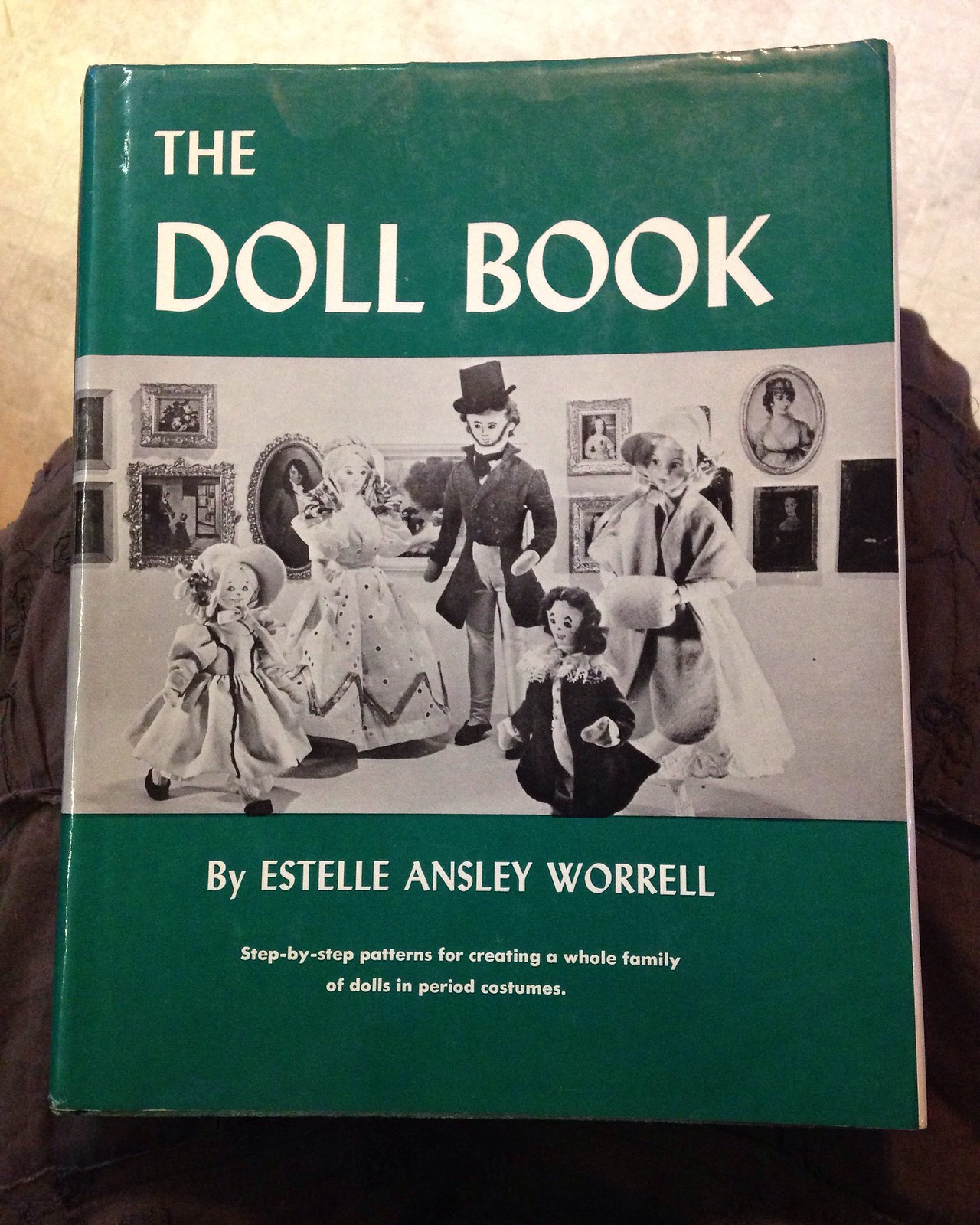The photograph depicts an old paperback book with a dark green cover. Prominently displayed at the top in large, uppercase bold white letters are the words "The Doll Book." Centrally positioned on the cover is a black-and-white photograph of five dolls dressed in vintage attire, resembling styles from the 1800s or early 1900s. These dolls are arranged as if gathered together, with detailed features: the one on the far left wears a white hat and black shoes; a centrally located doll resembles Abraham Lincoln with a black suit top, gray pants, black shoes, and a black top hat; other dolls show similar period-specific detailing in their attire. The backdrop of the photo includes several old, gray-scale portraits hanging on a wall, predominantly featuring people. Beneath this photograph, in white text on a green background, is the author's name, "By Estelle Ansley Worrell," followed by the subtitle, "Step-by-step patterns for creating a whole family of dolls in period costumes." The background setting where the book is placed includes a black fabric, possibly from the lap of a person holding the book, and a floor that appears white or yellow.